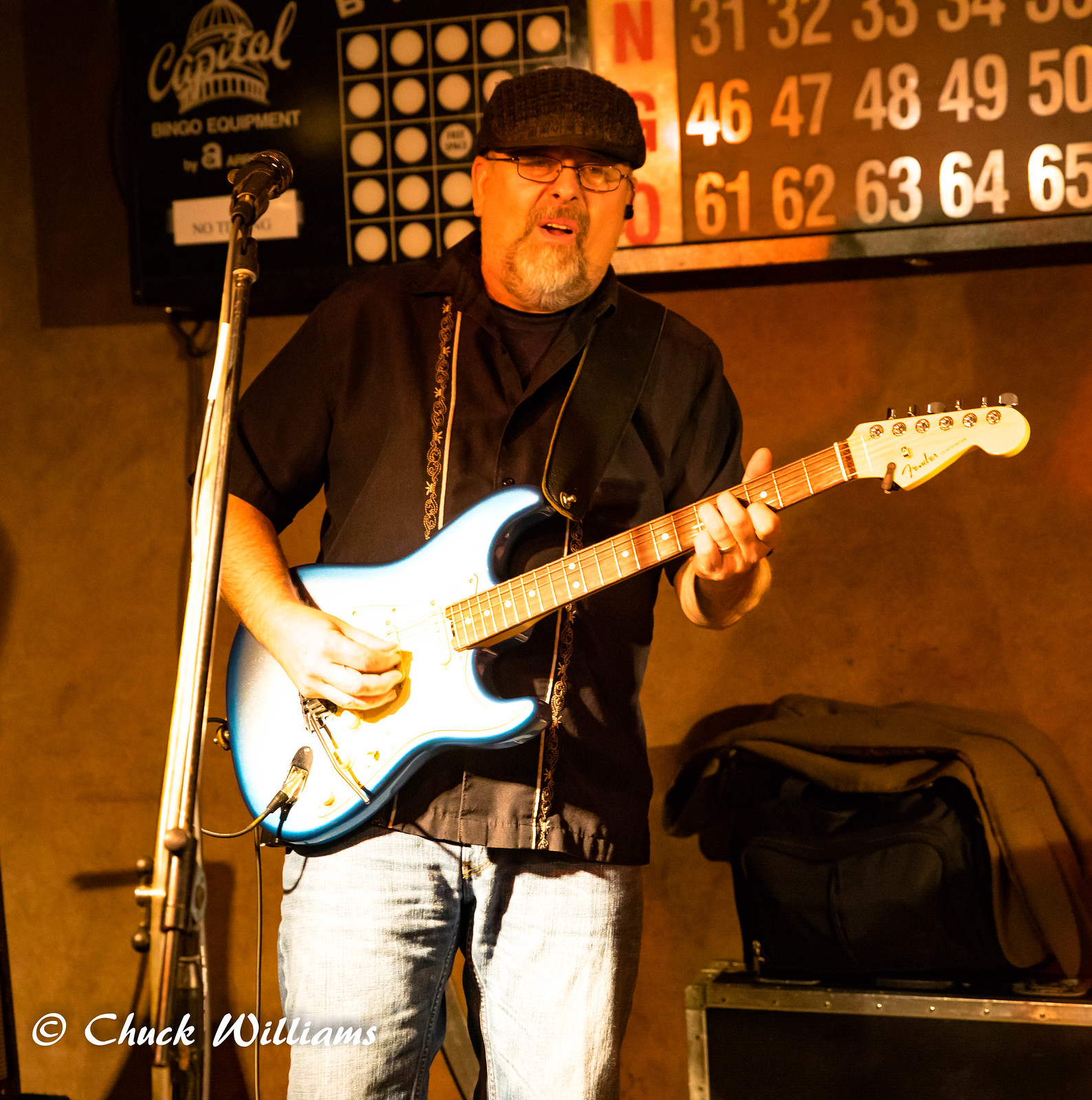The photograph captures a gentleman performing on a stage set against a brown background with bingo numbers displayed on a board behind him, indicative of a bingo hall. The man, appearing to be in his late 50s to early 60s, has a stocky build and wears wireframe glasses, a black beret-style hat, and a black shirt adorned with gold detailing stripes. He sports a graying beard and mustache. He is dressed in light denim blue jeans and is holding a distinctive blue Fender Stratocaster guitar, featuring a woodgrain pattern transitioning to blue at the bass. A microphone stands prominently before him, suggesting he is singing. At the bottom right of the image, a bag rests on what appears to be an amplifier. The bottom of the photograph bears the copyright mark "Chuck Williams," and at the top, the name "Capital Bingo Equipment" can be discerned, further affirming the setting.